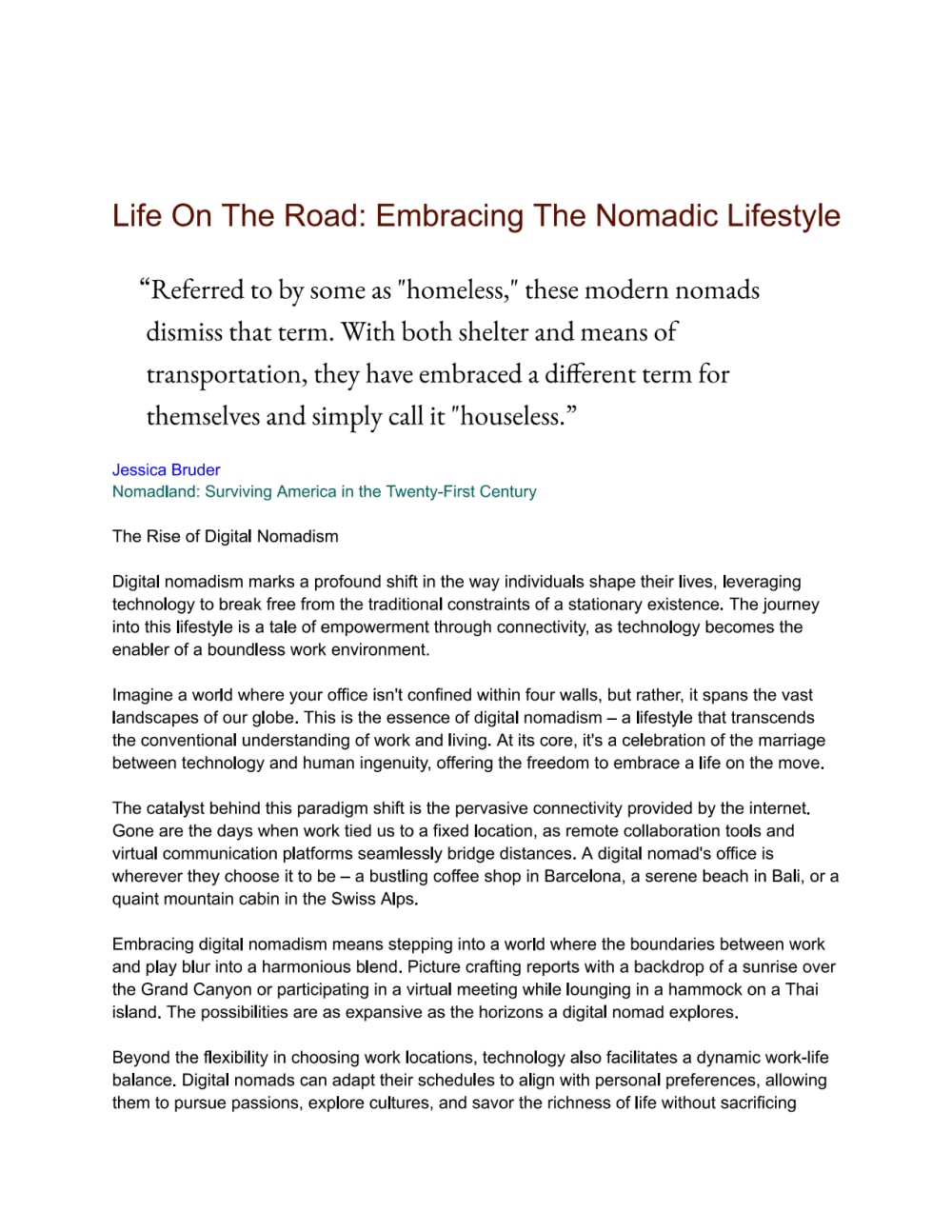The image displays an excerpt from an article titled "Life on the Road: Embracing the Nomadic Lifestyle" by Jessica Bruder. The page features a quote from the article about modern nomads, who prefer the term "houseless" over "homeless," emphasizing their unique lifestyle. Beneath the title, a subheading reads "Nomadland: Surviving America in the 21st Century." The visible portion of the article begins with the section "The Rise of Digital Nomadism," discussing the impact of technology on this lifestyle. The text describes digital nomadism as a transformative way of living, leveraging technology to break free from traditional work constraints and enabling a flexible, location-independent setup. Examples given include working from diverse locations like a bustling coffee shop in Barcelona, a scenic beach in Bali, or a mountain cabin in the Swiss Alps. The passage highlights how this lifestyle blends work and leisure seamlessly, offering a profound work-life balance. Note that the image captures only a portion of the article, ending abruptly mid-sentence. The text predominantly appears in black, with notable elements in blue and green, and some additional Korean writing at the bottom.